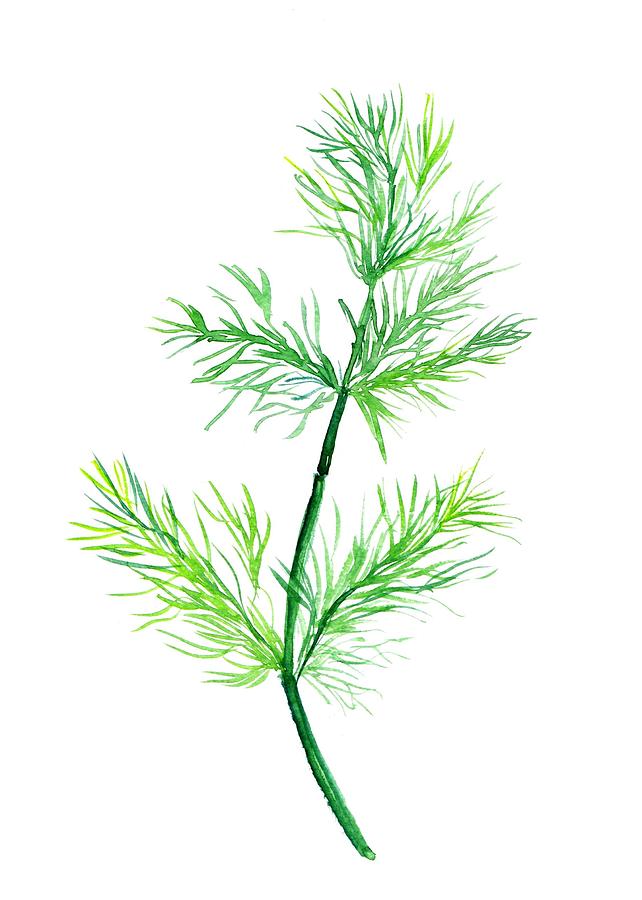The image is a detailed painting of a young pine or evergreen plant set against a completely white background. The plant features a curving green stem that extends from the bottom to the top of the image, transitioning in color from light green to dark green. Along this stem, tiny slivers of pine needle-like leaves branch out in five sections. These branches showcase a mix of light green leaves interspersed with darker hues and occasional yellowish tints, giving a watercolor effect. The leaves appear delicate and vibrant, especially towards the edges. The painting culminates at the top with clusters of light green needles pointing upward, suggesting a budding growth into a cone or triangular shape. The overall composition is precise and intricate, capturing the youthful, tender stages of the plant’s development.